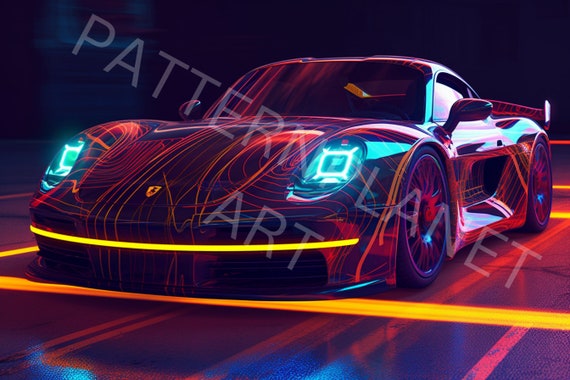This image showcases a digitally rendered, high-tech sports car that appears to be either a Ferrari or a Porsche, as indicated by the emblem on the front. The car presents a sleek, futuristic design in a deep purple color, adorned with vibrant, neon-hued swirls and stripes in oranges, pinks, reds, and blues. Its striking features include blue headlights with square halos, a bright yellow strip across the front bumper, and a spoiler at the rear. The car is depicted on a dark, black road detailed with fluorescent yellow lines and orange linear streaks, enhancing its cyberpunk aesthetic. The entire image bears a faint gray watermark that reads "Pattern Planet Art," hinting at its nature as a piece of digital or AI-generated art. The background is dark, making the vivid colors of the car and the road stand out prominently.